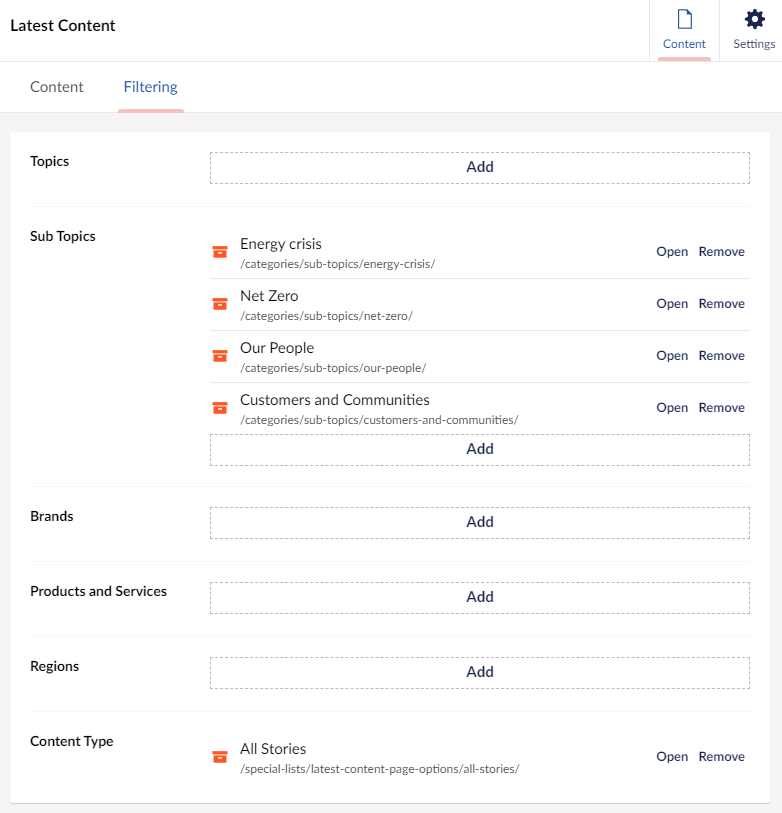The screen displays a web page interface with a clearly segmented layout. At the top, there is an empty topic screen labeled "Add." Below this, you find several subtopics including "Energy Crisis," "Net Zero," "Our People," and "Customers and Communities," each accompanied by a small red logo and options to open or remove the items. Proceeding downwards, a section titled "Brands" offers an add button, allowing users to include specific brands they wish to search for. Similarly, the "Products and Services" section provides an option to add relevant items. The subsequent heading is "Regions," followed by "Content Type" which lists "All Stories" along with a vaguely phone-shaped red logo and open or remove buttons. Underneath the "All Stories" section, additional categories such as "Special Lists," "Latest Content," and "Page Options" are listed, signifying a range of available content choices. The interface's general layout is unfamiliar, offering several customizable elements for user-specific content management.